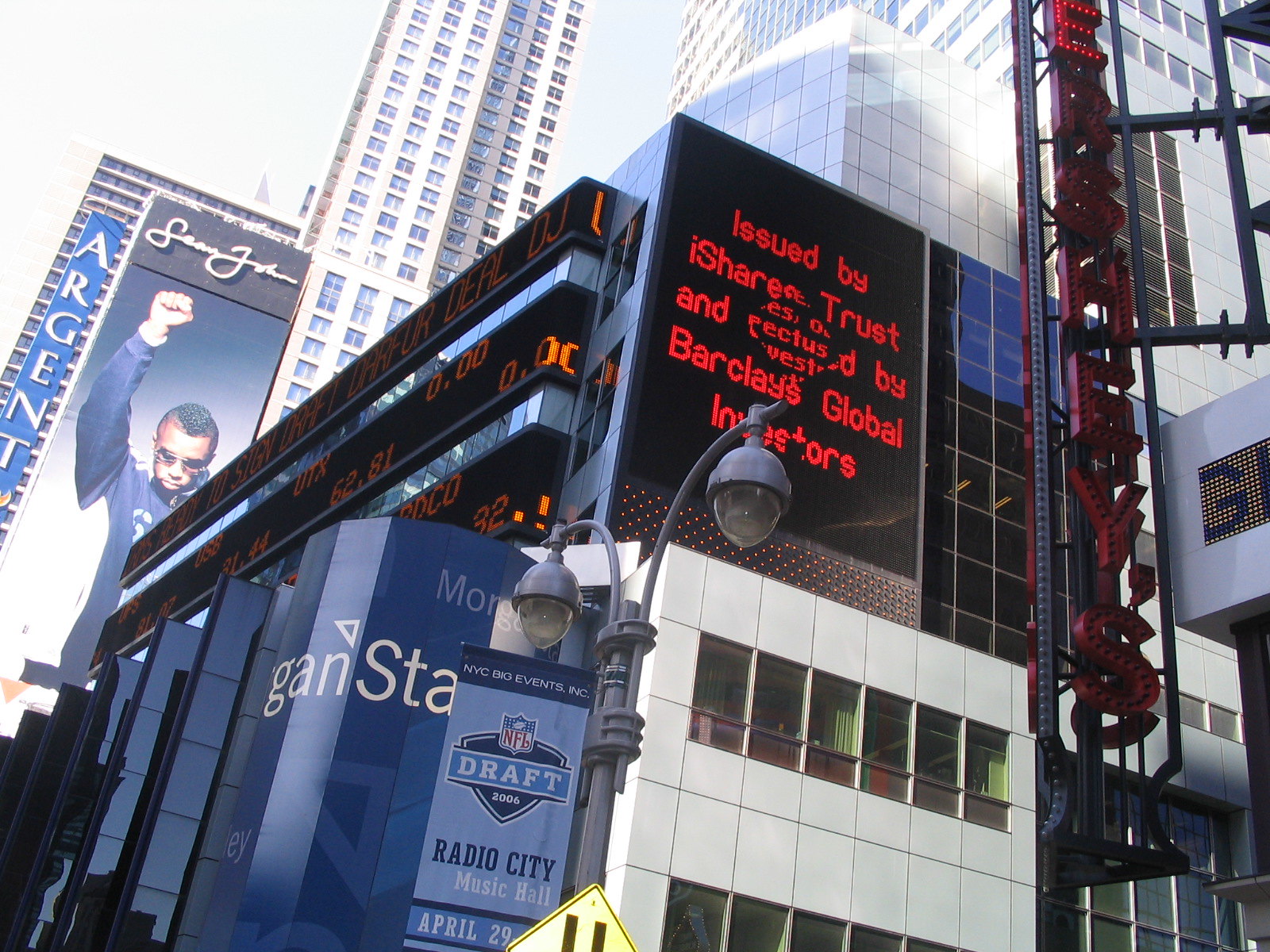A detailed cityscape captures a bustling daytime scene in New York City, dominated by towering skyscrapers that soar beyond the picture's frame. The focal point of the image is a large digital billboard emblazoned with red text, declaring "Issued by iShares Trust and by Barclays Global Investors." Nearby, a streetlamp with two hanging lights supports a vibrant banner that reads, "NFL Draft 2006 Radio City Music Hall, April 29th." The foreground is rich with reflective buildings featuring mirrored windows, while to the side, the Morgan Stanley building is prominently visible. In the distant background, the Argent hotel looms, complementing the scene with a striking image of a man raising his fist. The sky is a clear blue, adding to the urban grandeur. Various signs and banners contribute to the dynamic atmosphere of this downtown snapshot.